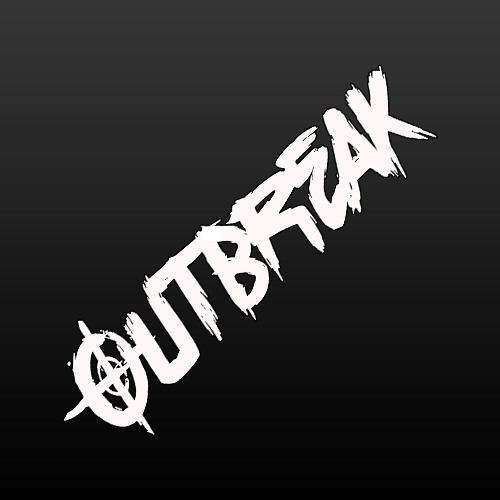The image showcases a bold, graphic design featuring the word "OUTBREAK" in all capital letters, set diagonally from the bottom left to the top right of a completely black background. The text is painted in white with a distinctive, dripping effect, giving it an unfinished, somewhat cartoony appearance. The letter "O" in "OUTBREAK" is designed to resemble a target, with an inner circle and a crosshair. This combination of stark black and white colors, along with the unique font style, suggests the image is likely a company logo or an advertisement, standing out vividly against the dark backdrop.